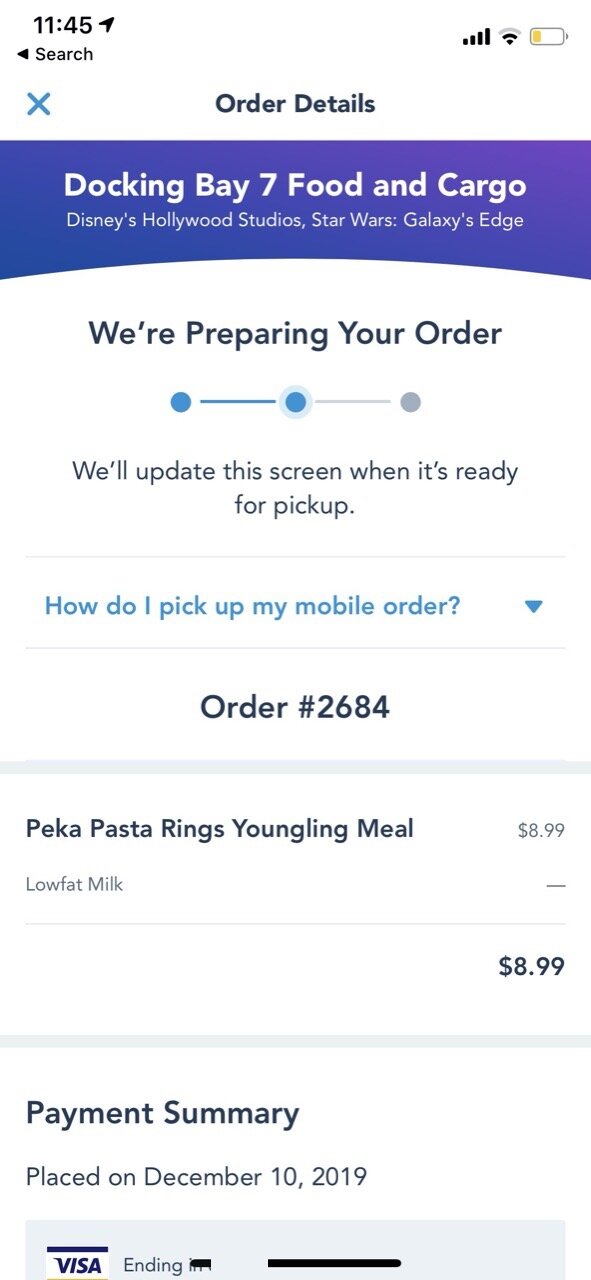The image depicts a mobile web page displaying the details of a recent order placed at Docking Bay 7 Food and Cargo, located in Disney's Hollywood Studios, within the Star Wars: Galaxy's Edge area. The page indicates that the order is being prepared and will notify the user when it's ready for pickup. The main portion of the screen is focused on an "Order Details" section that lists the order number (2684) and the items ordered. Specifically, the highlighted item is a "PEKA Pasta Rings Youngling Meal" priced at $8.99, which includes low-fat milk.

Additionally, there is a "How do I pick up my mobile order?" option that appears to be collapsible for more information. At the bottom of the page, the payment summary is shown, noting that the order was placed on December 10, 2019. The payment method is a Visa card, although the specific card details are obscured for privacy. Overall, this image captures the checkout page for a children's meal ordered within the Star Wars-themed section of Disneyland.